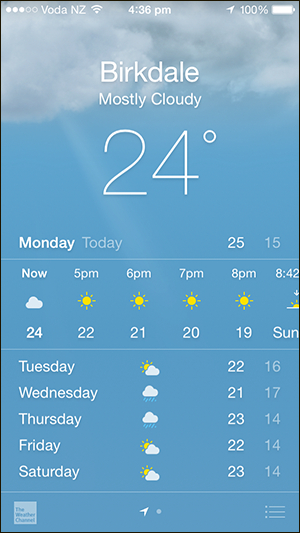A smartphone screen displays a weather application amidst a backdrop of a partly cloudy sky. At the top of the screen, three solid white dots and two outlined circles appear on the upper left corner, adjacent to the Wi-Fi indicator showing full connection. The status bar also displays the time as 4:36 p.m. and a fully charged battery icon, denoted as 100%.

Below, the weather app shows the location "Birddale" with a current condition of "Mostly Cloudy" and a temperature of 24 degrees. The weekly forecast highlights Monday in bold with a high of 25 degrees, followed by Tuesday with a high of 15 degrees. The daily forecast continues horizontally with graphical representations of clouds and sun, detailing temperatures at various times: 24 degrees at 5 p.m., 22 degrees at 6 p.m., 21 degrees at 7 p.m., and 19 degrees at 8 p.m., with a sun icon indicating sunset at 8:42.

A horizontal white line separates the days of the week, with temperatures listed for each day: Tuesday through Saturday, showing highs of 22, 21, 22, 23, 16, 17, and lows of 14 consistently through the latter end of the week. The comprehensive display gives a clear, detailed view of the weather predictions, allowing the user to plan accordingly.